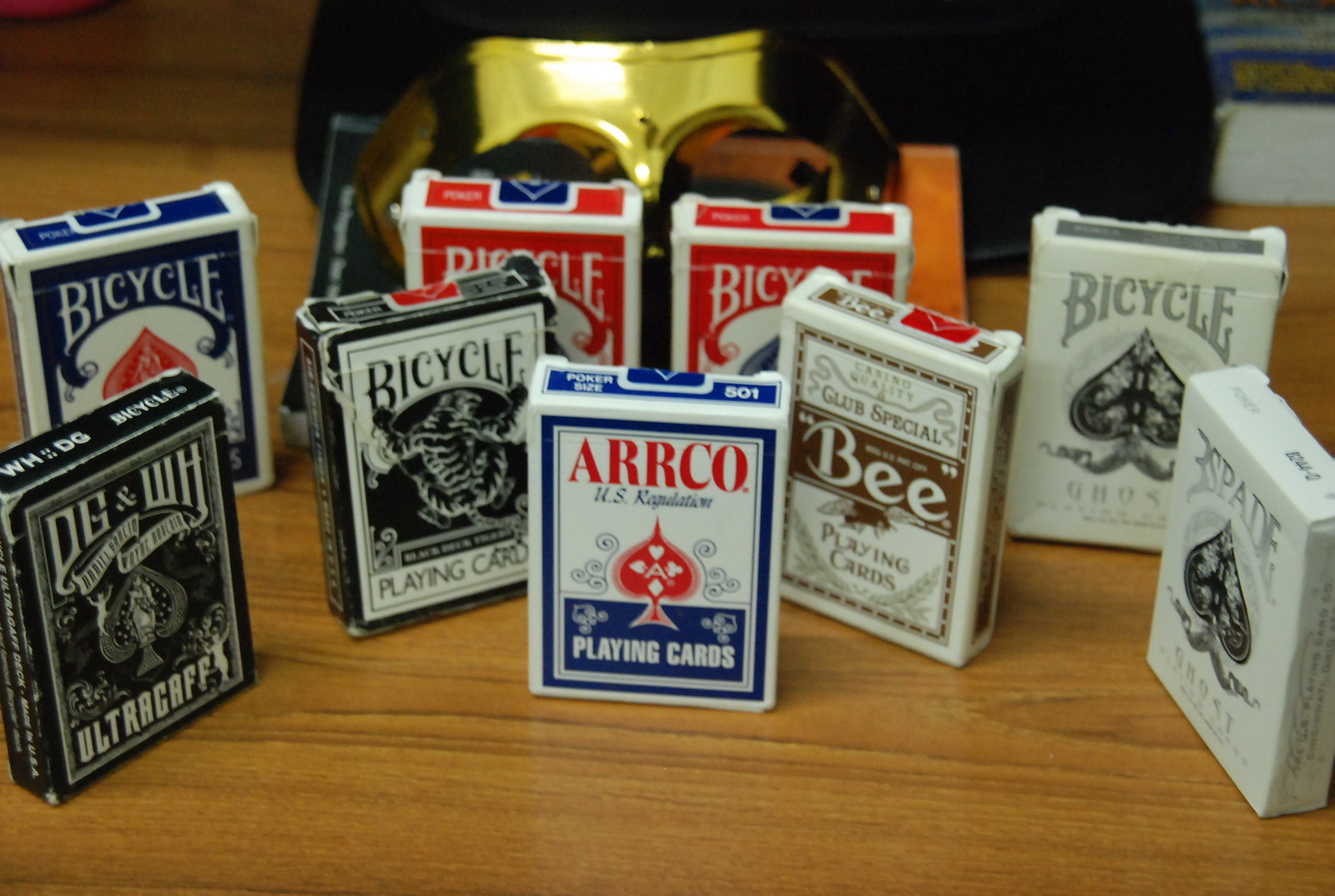In this photograph, several decks of playing cards are neatly arranged in their boxes on a table, showcasing a variety of designs and colors. On the far right, a box labeled "Bicycle: Ghost" in white, gray, and black features a prominent spade icon. Adjacent to it is another similar box with the word "Spade" and "Ghost" displayed on the bottom. A distinct brown and white deck labeled "Bee Club Special Playing Cards" adds to the diversity.

Towards the back, two red Bicycle card decks are visible, each stamped with a blue seal. However, the intricate decorations on these decks are not clear. Centrally positioned at the front is a white deck labeled "ARCO U.S. Regulation Playing Cards," adorned with a red spade on its face. Another intriguing deck, in black and white, is marked "Bicycle Playing Card" and features an image of what appears to be a monster in the middle.

Additionally, a blue Bicycle deck also garnished with a red spade, and another black and white deck labeled "WHDG Bicycle" with the words "Ultra Cafe" partially readable at the bottom, are present. 

In the background, an unusual yellow object with eye openings—resembling a helmet or glasses—adds a mysterious element to the scene, with hints of orange visible within.